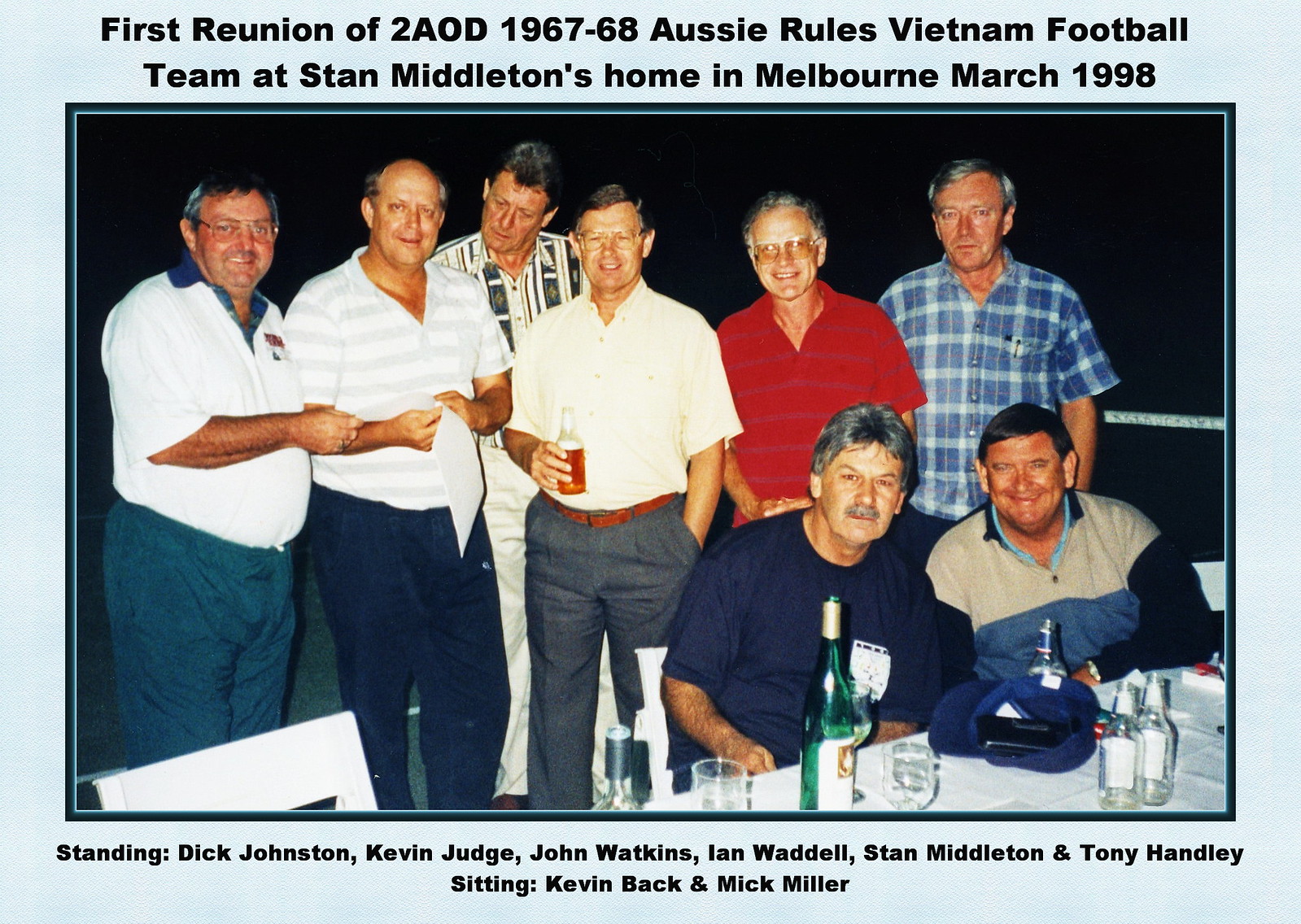In the image, eight older gentlemen are gathered at what appears to be a professional photograph taken during the first reunion of the 2A OD, 1967-68, Aussie Rules Vietnam football team at Stan Middleton's home in Melbourne, March 1998. The picture features a distinct light blue border that frames the entire scene and displays the event's title and date at the top. Six of the men are standing in the center of the image, while two are sitting at a table in the front foreground. The men are dressed in slacks and a mix of dress-up polos and flannel shirts.

The table in front of the seated men holds an assortment of liquor bottles, beer bottles, and wine bottles, along with glasses, suggesting a convivial atmosphere. The setting behind them appears to be nighttime, as it is black outside. All the men have gray hair, and several are wearing glasses—specifically, the first man on the left and the second man to the right. One of the seated individuals sports a mustache, adding to the varied appearances among the group. They are all smiling, capturing a moment of happiness and camaraderie. Beneath the image, their names are listed: standing are Dick Johnston, Kevin Judge, John Watkins, Ian Waddell, Stan Middleton, and Tony Hanley; sitting are Kevin Beck and Mick Miller.